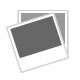This detailed image shows a rectangular warning sign placed on a white, square table with curved edges. The sign, white with a black string tied for hanging, prominently features a black-and-white illustration of a skull and crossbones. The eyes and nose of the skull are shaded in black ink, and a red, zigzag arrow is drawn from the top of the skull and extends through the bottom of the crossbones. Surrounding the illustration, there is text written in what appears to be a foreign language—likely Germanic or Slavic—ending with the word "ELEKTRYCZNE," suggesting a warning related to electricity.